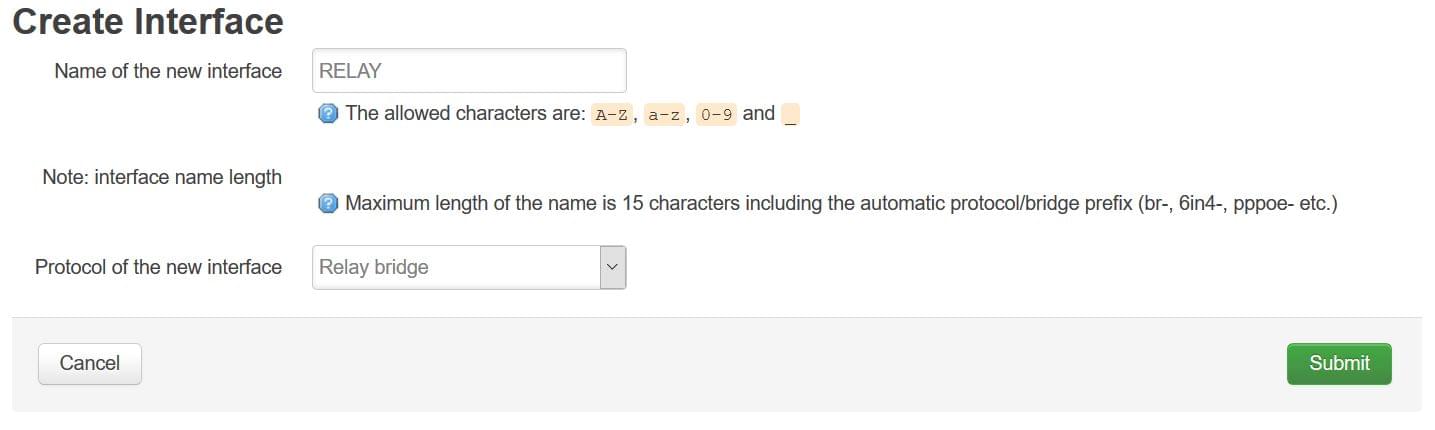The image displays the "Create Interface" section positioned at the upper left-hand side, prominently marked with bold font. Beneath this header, the text "Name of the New Interface" is visible, followed by a light gray square containing the word "Relay." Below this, there is a specification regarding allowed characters, stating: "The allowed characters are A to Z (capitalized), a to z (lowercased), 0-9, and underscore (_)." 

Further down, a note indicates: "Interface Name Length," explaining that the maximum length for the interface name is 15 characters. This length must include the automatic protocol/bridge prefix—such as _BR-6IN4, -PPPoE, etc.—in the character count. 

The section also features a search bar at the bottom where users can search for the protocol of the new interface.